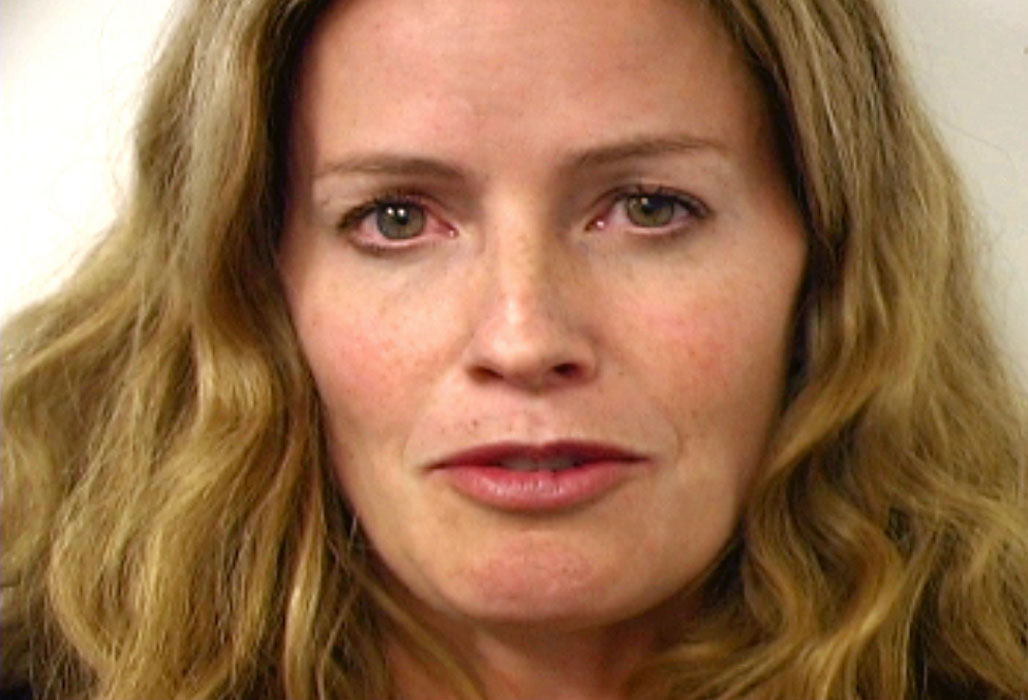The image is a detailed portrait of a middle-aged woman standing against a white background. Her long, wavy blonde hair cascades around her neck and under her chin, hiding her shoulders. She has green eyes that are slightly red, as if she has been crying, with her right eye appearing more affected than the left. Her delicate features include a thin top lip, a small nose, a square chin, and flushed cheeks, possibly accented with a bit of blush. She wears very little makeup, except for some mascara on her eyelashes and a hint of pinkish-red lipstick on her lips, which are slightly open in a subtle, almost melancholic smile. Her brows match the color of her hair and frame her lightly freckled face. The overall expression on her face is one of sadness or deep concern, highlighting the emotional tone of the portrait.